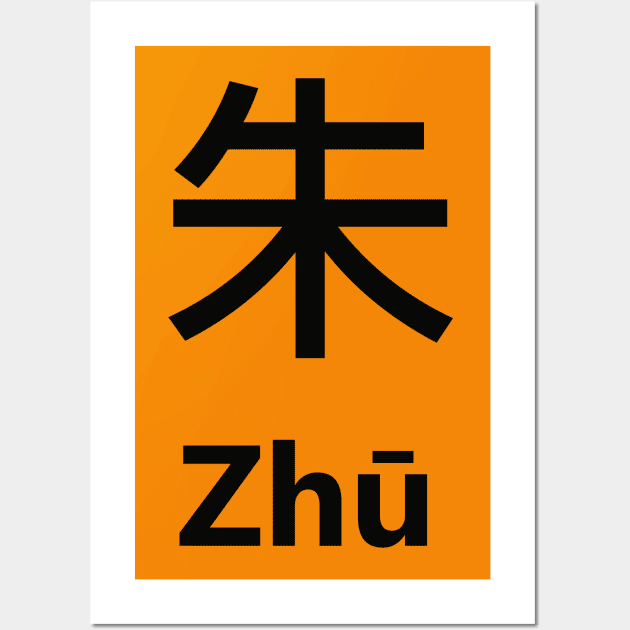This image features a vertically oriented rectangular sign centered against a gray background. The sign is divided into two main segments: an inner segment featuring a vibrant orange background resembling canvas, and an outer segment with a white border. 

At the top of the sign is a large, prominent Asian character. Below this symbol, the word "ZHU" is displayed in black font, with a macron (a horizontal line) over the "U" to indicate its pronunciation. The detailed design and color contrast between the black text and orange backdrop make the symbols and their explanation discernible and visually striking.